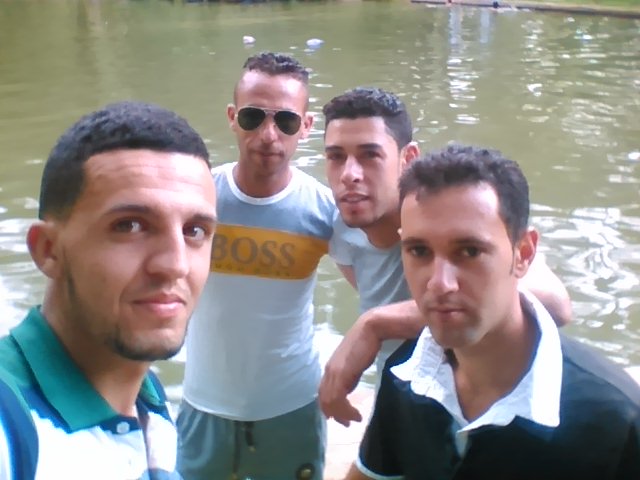This full-color outdoor photograph, taken during the daytime, features four young men standing close together, looking towards the camera as if posing for a photo. The man on the left appears to be taking a selfie. All four have short dark hair, with three of them clean-shaven and one sporting a slight beard. One man is wearing sunglasses, while the others are not. They are all dressed in short-sleeved shirts; the two men in front wear three-button collared polo shirts, and the two in the back wear t-shirts, with one of the t-shirts displaying the word "boss."

The background showcases a calm, relatively murky body of water, likely a pond or lake, with visible sun reflections dappling the surface. On the far upper right, there is a glimpse of the shoreline. The colors in the image include blue, green, white, gray, brown, black, and yellow. Subtle reflections of trees or tree trunks can be seen at the top part of the image on the left side. The overall setting appears to be a comfortably warm day, inferred from the casual, summery attire of the men.